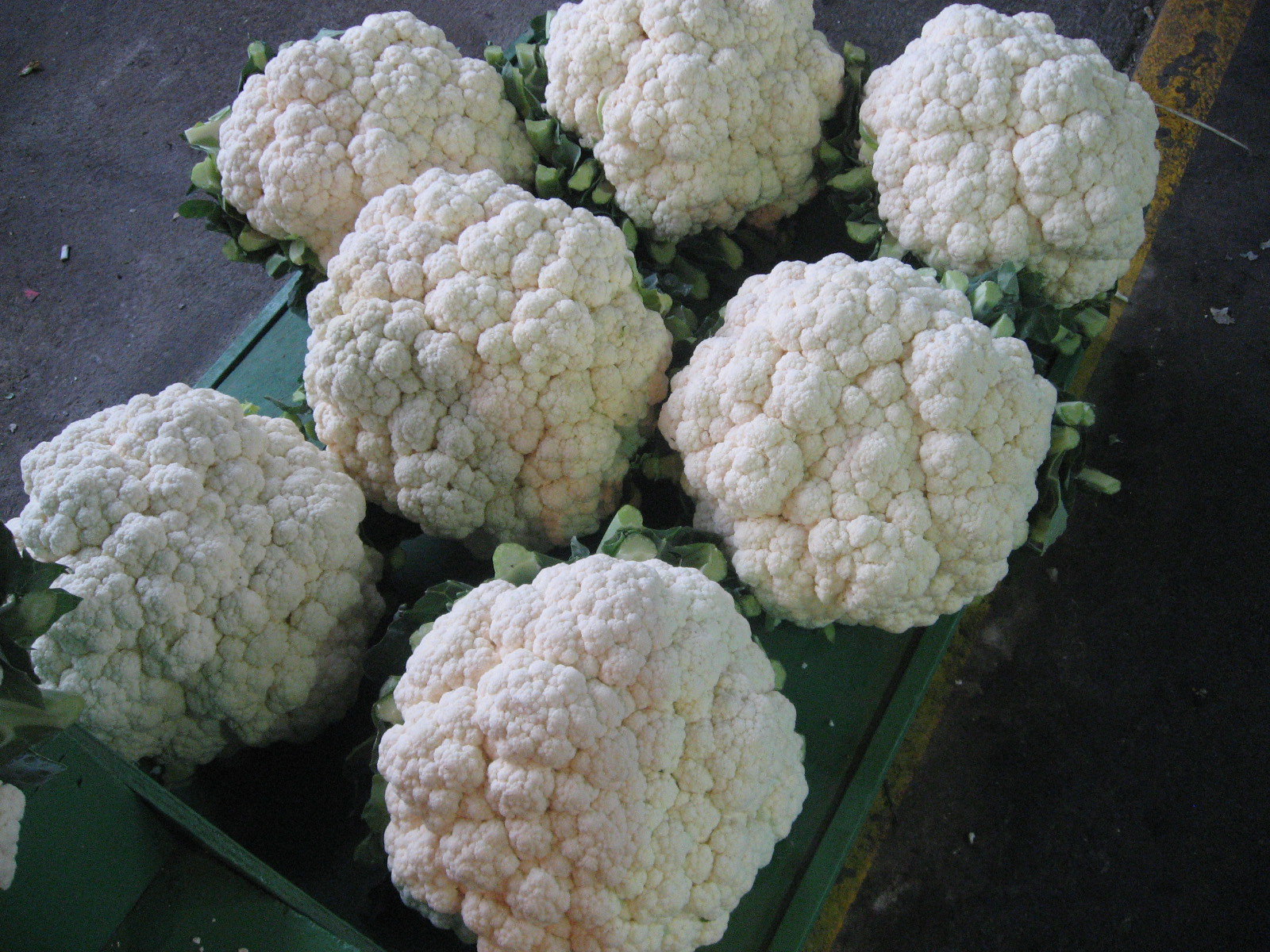This photograph captures a top-down view of seven large, fluffy white cauliflower heads arranged on a dark green wooden stand or crate. The cauliflower heads are prominently displayed with their light green stems and dark green trimmed leaves peeking from underneath. The backdrop appears to be an asphalt street, marked by a partially scrubbed-off yellow line running from the upper right to the bottom right middle, suggesting the edge of a road. The vivid contrast between the bright white cauliflower, the green leaves, the dark green stand, and the textured asphalt creates a striking and detailed composition.